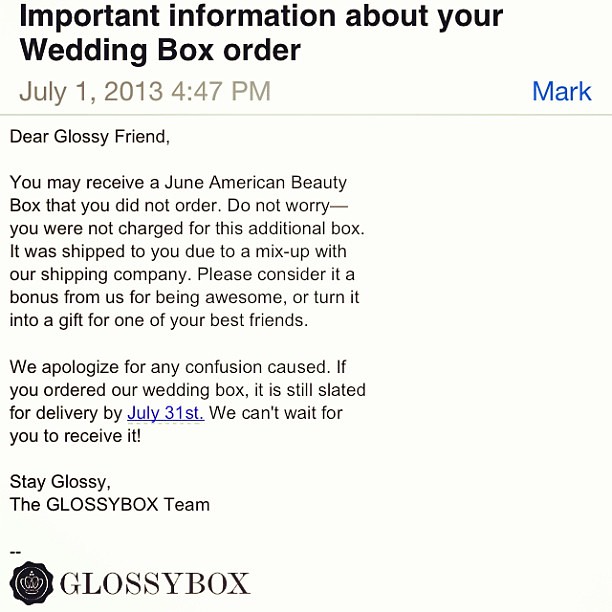The image shows a screenshot of an email from Glossy Box, viewed on what appears to be an iPhone. The email, on a white background with black and grey text, is titled in bold, “Important information about your wedding box order.” Directly below, in grey text, it reads "July 1, 2013, 4:47 PM," with the name "Mark" in blue text to the right. A horizontal line divides the header from the email body, which starts in smaller black text: “Dear Glossy Friend, You may receive a June American Beauty box that you did not order. Do not worry, you are not charged for this additional box. It was shipped to you due to a mix-up with our shipping company. Please consider it a bonus from us for being awesome, or turn it into a gift for one of your best friends. We apologize for any confusion caused. If you ordered our wedding box, it is still slated for delivery by July 31. We can't wait for you to receive it.” Notably, “July 31” is in blue and underlined, resembling a hyperlink. The email concludes with, “Stay Glossy, The Glossy Box Team.” At the very bottom, there's a black insignia resembling a stamp with a crown, accompanied by the text “Glossy Box.”